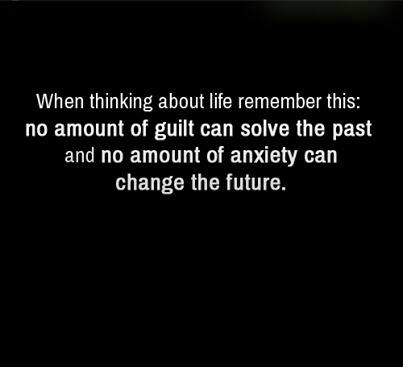The image features a solid black background with white, center-aligned text, positioned slightly towards the upper half. The text reads: "When thinking about life, remember this. No amount of guilt can solve the past, and no amount of anxiety can change the future." This motivational message is designed to be shared on social media or used as an informational piece or poster. The phrases "no amount of guilt can solve the past" and "no amount of anxiety can change the future" are emphasized in bold, adding visual weight to these key points. The overall composition is simple yet impactful, delivering a powerful reminder about focusing on the present.